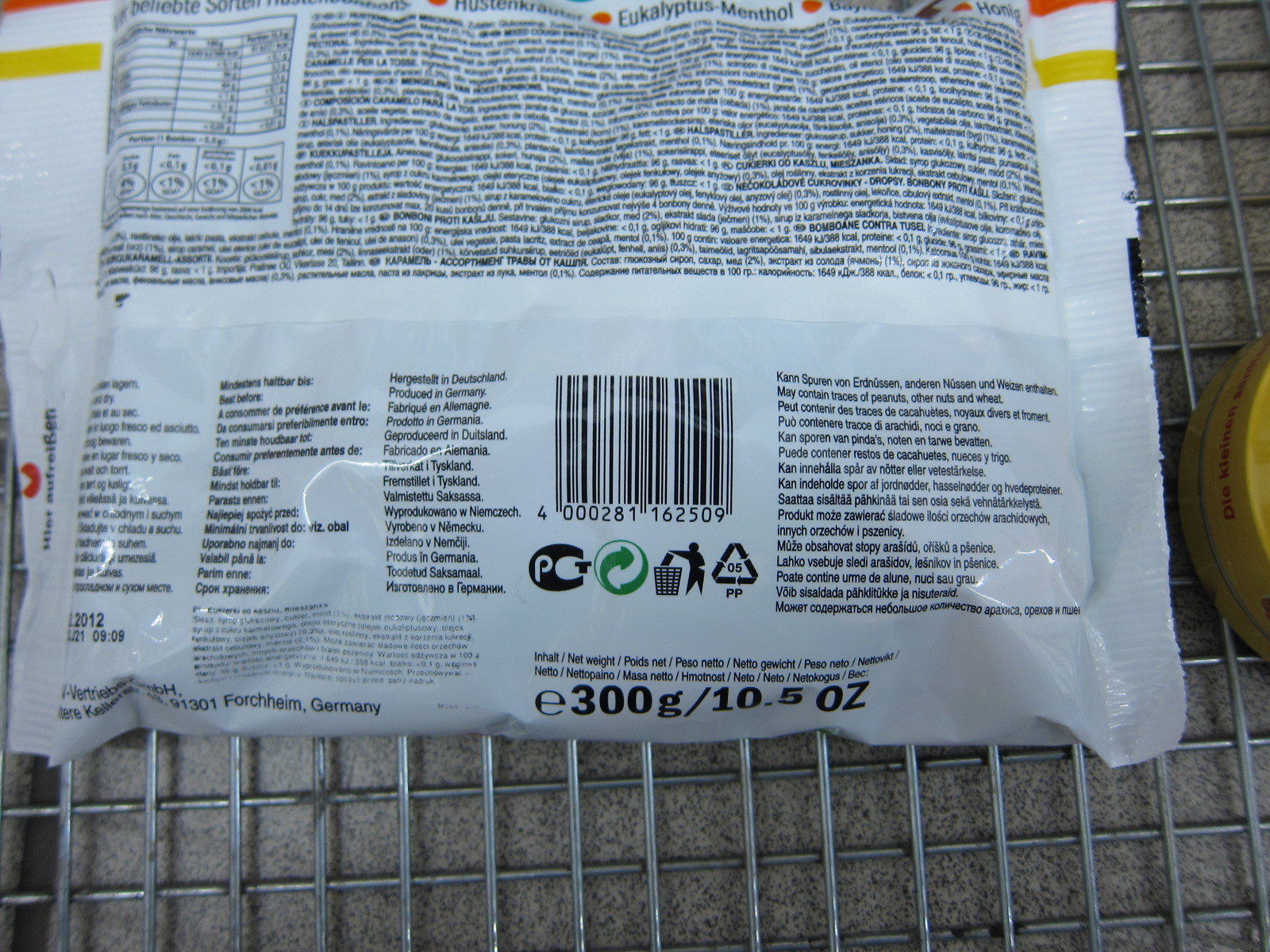An indoor color photograph taken from above shows a plastic food package resting on a metal or chrome grid surface. This setting suggests that the package is either in a refrigerator or on a shelf in a supermarket. The photograph focuses on the back of the package label, which is predominantly covered in fine print text that appears out of focus.

The upper half of the label is entirely filled with black fine print text, while the lower half also contains fine print text, mostly out of focus as well. Near the right center of the label, the barcode is visible with the number "4000281162509" clearly displayed below it. Just below the barcode, a series of symbols are visible. To the immediate right of the barcode is a black "C" symbol. Next to it is a yin-yang symbol in white and green. Following this is a silhouette of a person putting an item into a trash can. On the far right, there is a rectangle containing the number "05" above the letters "PP."

Additionally, the weight of the package is clearly indicated at the bottom of the label as "E300G / 10.50OZ." Despite the detailed view of the label, no specific information about the contents of the package is discernible. It is a plastic food package likely containing an unidentified food item.